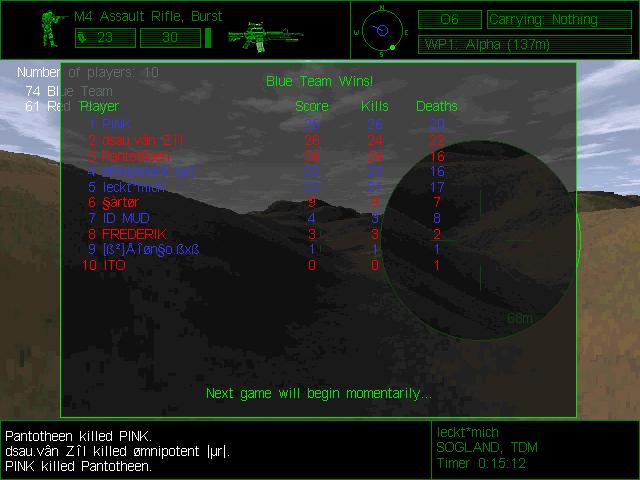The image captures a screenshot of a military-themed video game, featuring a desert landscape in the background overlaid with various gameplay stats and player information. The top left of the screen shows a small icon of a military man and the text "M4 Assault Rifle Burst" alongside an image of the weapon. The upper part of the screen displays numerical stats, such as "23 30" and "WP1 Alpha 137M," while the middle of the screen prominently declares "Blue Team Wins" in green text. Following this, game statistics including scores, kills, and deaths are presented, likely in multiple colors including red for specific game scores. The lower portion of the screen notes, "Next game will begin momentarily," and includes a running commentary of player actions such as "pantothene killed pink" and complex alphanumeric names like "I-D Mud" and symbols. Additionally, the players' names—some of which are not clearly identifiable or are symbol-based, such as "A-R-T" with an unknown character and "Frederick"—appear on the left side of the screen. The timer in the bottom right corner reads "0:15:12," indicating the time elapsed or remaining.